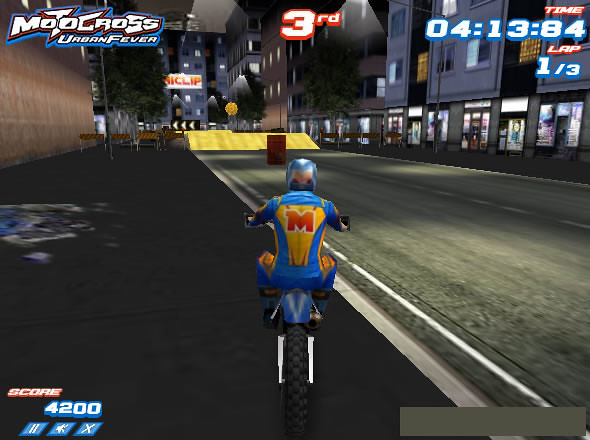The image is a screen capture from the video game "Motocross Urban Fever," as indicated by the logo in the top left corner. The scene takes place on a city street at nighttime. The player, positioned in the center foreground and viewed from behind, is riding a motorcycle with distinctive black tires. The rider is clad in a blue riding suit with yellow highlights and a large red "M" on the back, and equipped with a blue helmet. Various game stats are displayed around the edges: the player is currently in third place (indicated in red text at the top center), the timer in the top right shows 4 minutes, 13.84 seconds, and they are on lap 1 out of 3. The score in the bottom left corner is 4200, accompanied by a pause button, a speaker icon, and an 'X' button. The city street background features storefronts on the right-side buildings and a large brown wall on the left. Yellow ramps and a red barrel are visible ahead of the player on the road, adding elements of challenge and excitement to the scene.